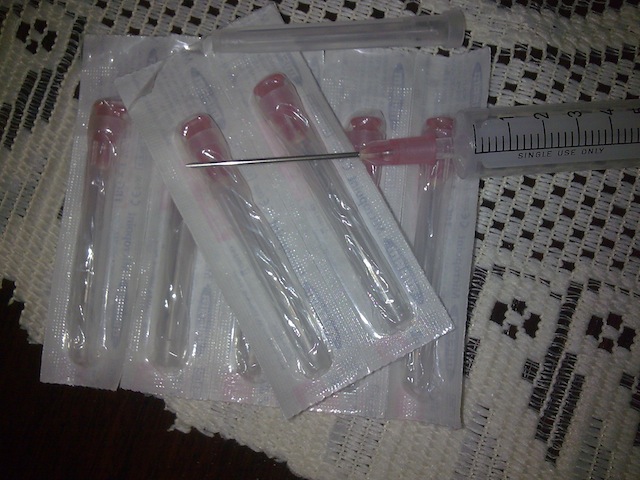The image showcases a close-up scene, possibly taken inside a home, where a syringe and its accessories are meticulously arranged on a textile surface. Central to the image is a standard, single-use, translucent syringe featuring graduation markings and the text "single use only" in black. The syringe, complete with a sharp needle and a pink tip, lays horizontally across several sealed packets. These packets, which appear to contain additional syringe tips or needles, are wrapped in clear plastic and organized in pairs. The entire setup is placed on a detailed, woven white doily with black and gray stripes and dots, which serves as a decorative table covering atop what looks like a black table. Additionally, a detached needle cover can be seen resting above the packets.